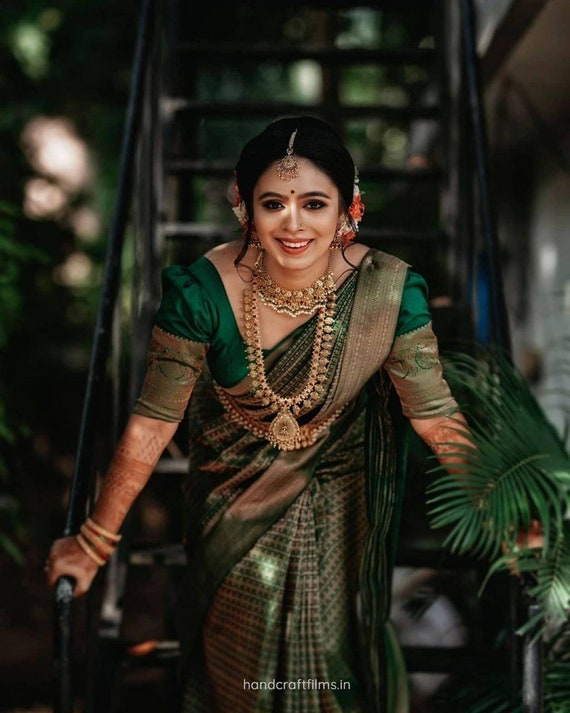This photograph depicts a beautifully adorned Indian woman standing gracefully on the bottom step of an outdoor black metal staircase, with a lush green background and a palm bush partially obscuring one of her hands. She is strikingly dressed in an emerald green and gold sari, accentuated by intricate henna designs that extend up her arms almost to her elbow. Her elaborate jewelry includes a heavy double-part necklace—one section like a choker and another hanging down with a medallion and dangling strings, mirroring the ornate jeweled headpiece with additional strings on her forehead, which is marked by a traditional bindi. Her ensemble is complemented by bracelets and possibly a hint of flowers in her upstyled dark hair, which features a few tendrils gracefully framing her smiling face. The backdrop is daylight-lit, though slightly blurred, emphasizing her radiant and meticulously crafted appearance. The image bears the watermark "handcraftfilms.in," suggesting it might be a stock photo representative of Indian cultural attire.